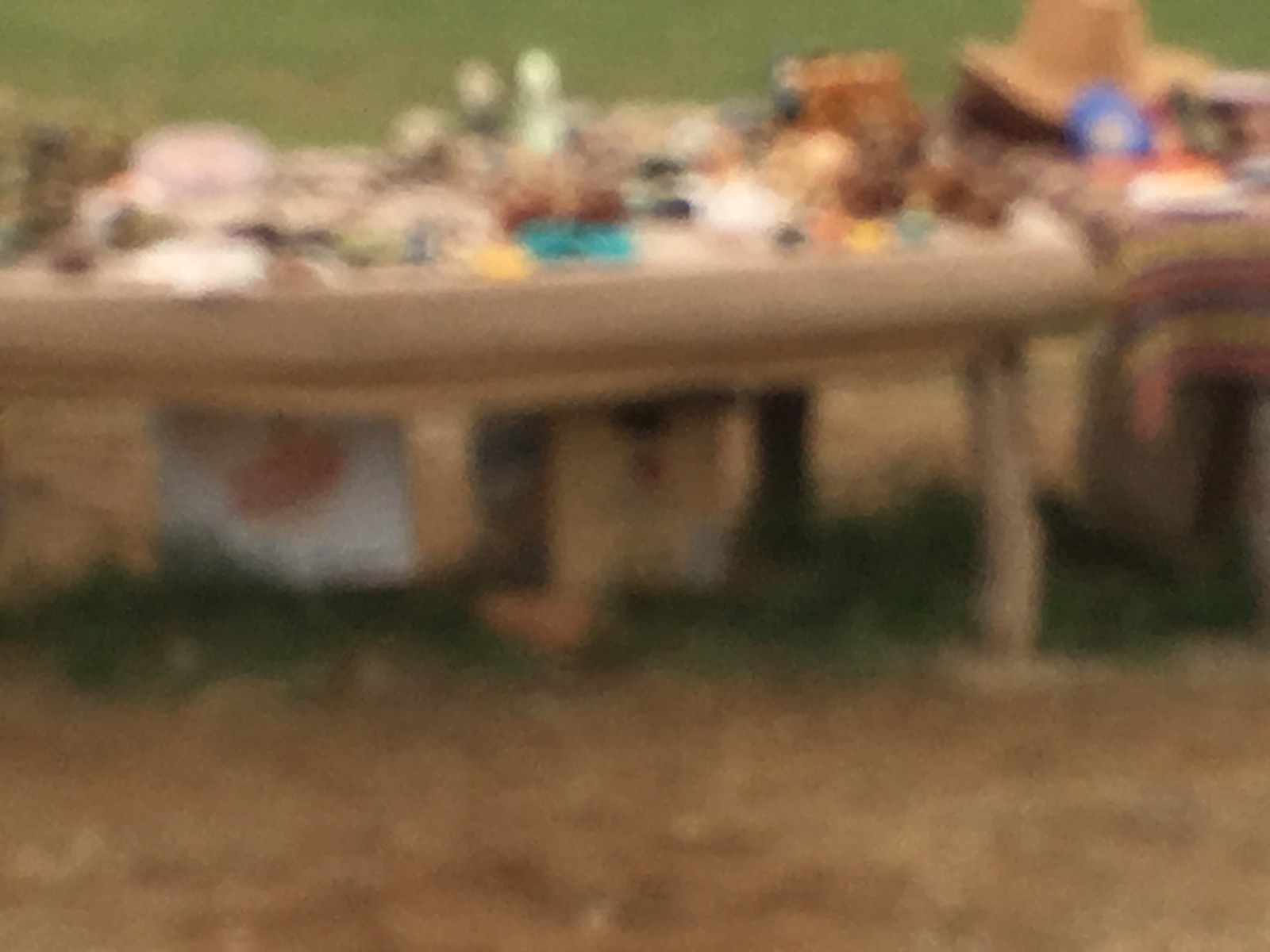This image is very blurry, making it difficult to clearly discern details. The setting appears to be outdoors, as the ground beneath and around a table is grass. Notably, much of the grass is dead and brown except for a green patch directly under the table, suggesting it has been shielded from sunlight. The table itself seems to be made of light wood and is irregularly shaped, with a possibility of an additional table beside it. Both tables are covered with assorted, indistinguishable items, which might include knickknacks and hats. On the right side of the main table, there appears to be a sombrero-like hat and some sort of table covering, possibly a striped blanket in yellow, red, and brown hues. There's also mention of a brown box and a white bag with a shape on it, adding to the assortment of items. This setting evokes an atmosphere reminiscent of a yard sale or flea market.